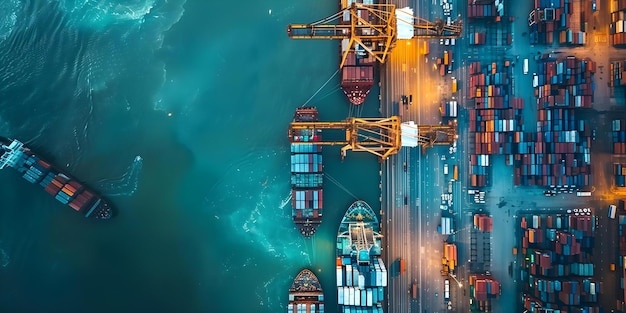This aerial, creatively rendered image displays a bustling port scene with a stunning photorealistic quality, albeit created digitally. Dominating approximately three-fifths of the left side of the image is a dark blue ocean, churning with swirling eddies and waves. In this waterway, five cargo ships are present, stacked high with an array of colorful metal freight containers in various hues of white, blue, yellow, orange, and brown. Four of these ships are neatly aligned parallel to the dock, while a fifth ship is depicted approaching the dock from the left edge of the image, creating ripples in the emerald green water as its wake is visible.

On the right-hand side of the image, the dock area is visible, paved and organized with an array of stacked cargo containers. These containers appear to be either awaiting loading or recently unloaded. Two large yellow cranes extend over the docked ships, actively loading or unloading the freight. There is also a road on this side, noted for appearing almost blue from this aerial or drone-like perspective. The lifelike scenery, captured in what appears to be daytime, vividly illustrates the dynamic operation of the port, efficiently handling global cargo shipments.